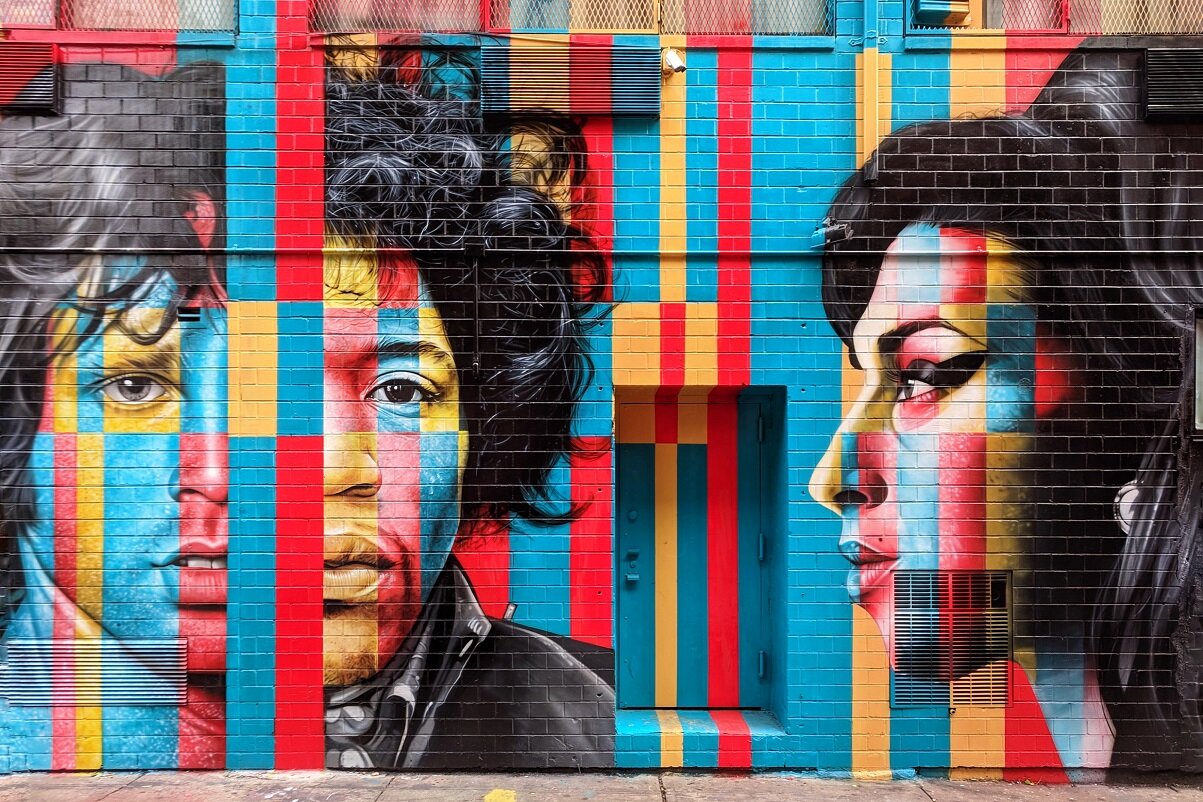The mural on the side of a brick urban city building is a captivating piece of street art. The right side features an unmistakable profile of Amy Winehouse, showcasing her iconic beehive hairstyle and distinctive eyeliner. The left side of the mural includes two other musicians, although less recognizable, depicted with half of their faces showing. One has long, wavy hair with facial hair, while the other has big, curly hair, and both are rendered in black and white. Across their faces are striking blue, red, and yellow squares and stripes, adding vibrant cross-sections of color to the artwork. The mural also includes a door in the center with a yellow vertical line and a white camera positioned above, looking down on the scene. The complex interplay of colors and figures makes this mural a striking and dynamic piece of urban art.